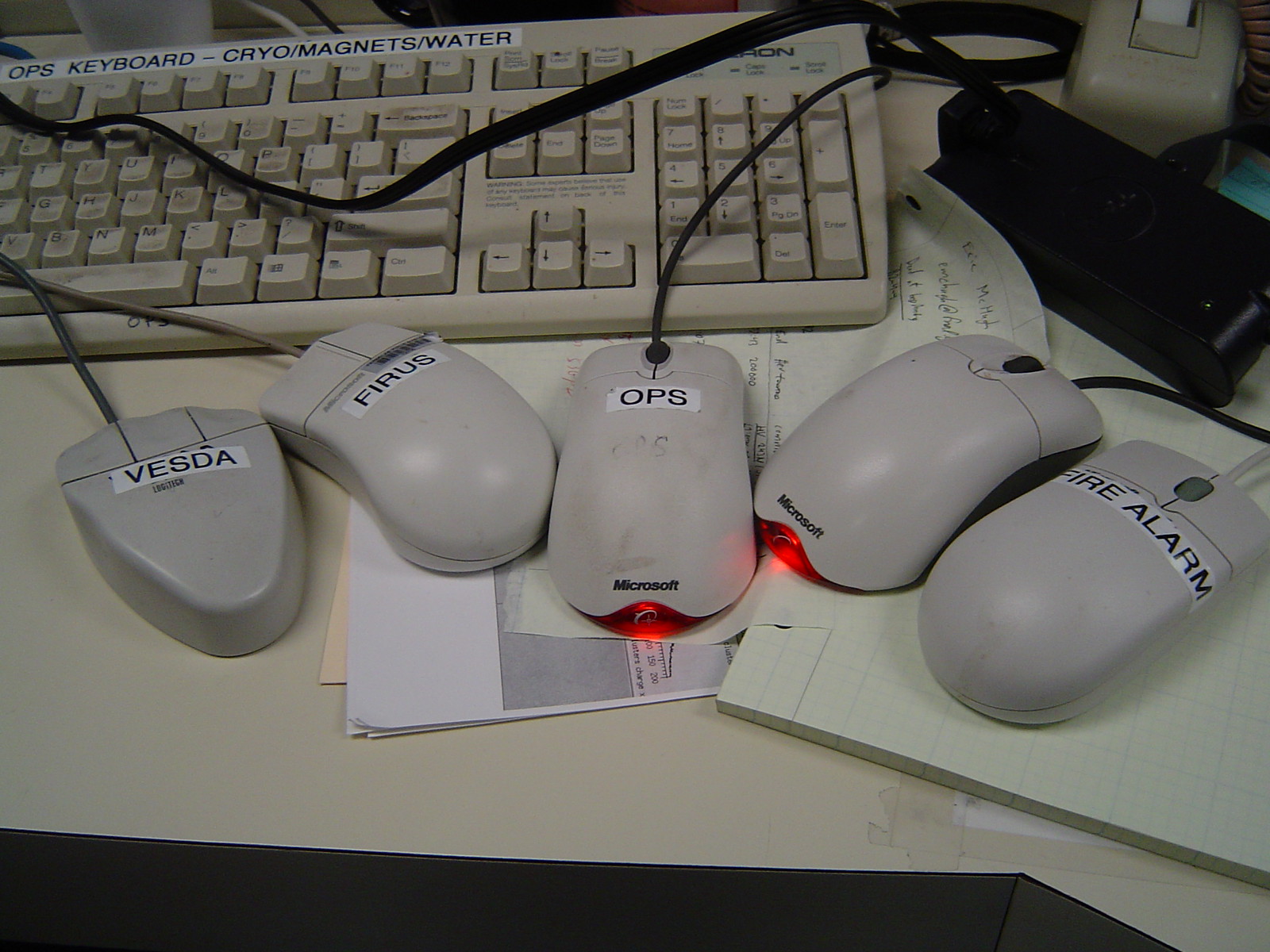This vintage top-down image appears to have been taken in the 90s or 2000s and features a corner desk with a creamy white or yellowish white surface with a dark border. On the desk lies an old-fashioned, bulky beige keyboard, adorned with a sticker that reads "OPS Keyboard - Cryo/Magnets/Water." This keyboard occupies the upper part of the image, with a black cord draped across it. Below the keyboard sits five computer mice arranged in a semi-orderly fashion, atop various sheets of paper, including yellow notepad paper and graph paper.

The mice are diverse in appearance, with distinctive shapes and varying levels of wear, indicative of their age. The leftmost mouse is V-shaped with three distinct buttons, labeled "VESDA" in black letters on a white sticker. Next to it, a more modern-looking mouse with two buttons bears the label "FIRUS." The middle mouse, rectangular and branded Microsoft, is marked "OPS." To its right, another square-shaped Microsoft mouse has no label. Finally, the mouse on the far right, also square-shaped with a significant hump towards the back, is labeled "Fire Alarm." Above the keyboard is a bulky power supply and a roll of gray tape, contributing to the cluttered, tech-heavy scene.